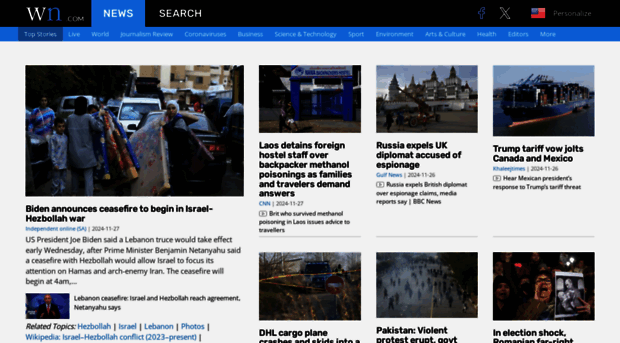The website displayed is "whitewbluen.com". Prominently featured is a navigation bar at the top with the site name in blue letters, with the center section reading "NEWS" and a black search bar extending across the right side of the page. Below that, an image of the American flag is shown with the word "Personalize" above a blue bar. Just beneath, a live news ticker streams various headlines, though the text is small and difficult to read.

On the left side of the page, a prominent headline reads: "Gaza War: Israeli Intel Warned of Hamas Plans Weeks Before October 7th Attack – Report." This section includes an image of soldiers in a battlefield and provides additional context about the conflict.

Further down, another headline reads: "Putin's Visit to Pyongyang Likely to Deepen Anti-Western Ties," accompanied by an image of two people shaking hands, presumably representing Russian and North Korean leaders.

There are also five other smaller news snippets with images. One article highlights, "Governor Wes Moore: Driven, Charismatic, and Maybe America's Future President." Another urgent headline says, "World Urged to Take Action to Enforce International Law in Middle East," featuring an image related to military conflict. A third snippet shows a picture of a nuclear warhead with a headline concerning nuclear issues, and another news piece warns, "Low Snow on the Himalayas Threatens Water Security: Study," featuring an image of the Himalayas.

Overall, the website layout is visually engaging but somewhat crowded with multiple headlines and images emphasizing current international news and significant geopolitical events.